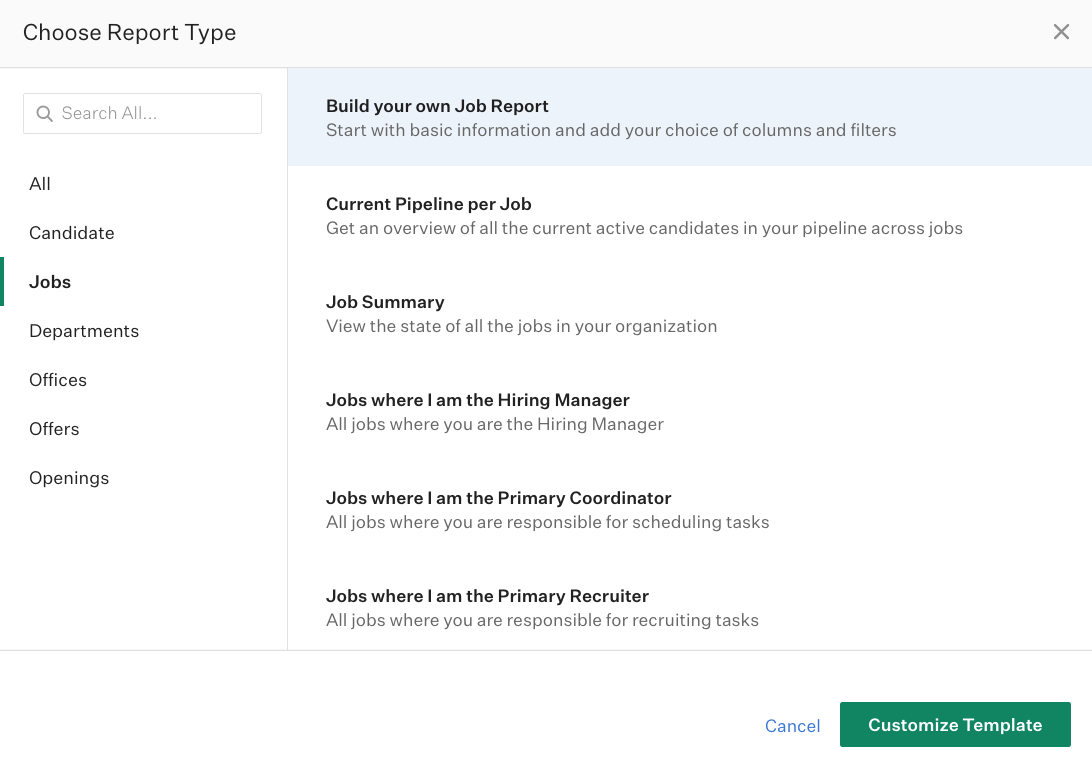The screenshot depicts a computer interface. At the top, a gray bar extends across the screen. On the left side of the bar, the text "Choose Report Type" is displayed, while the right corner features an 'X' icon for closing the page. Below the gray bar, the screen is divided into two main sections.

On the left-hand side is a panel with a search bar at the top. Beneath the search bar, a list of categories is displayed, including: "All Candidate Jobs," "Departments," "Offices," "Offers," and "Openings." The "Jobs" category is highlighted with a green line beside it, indicating it is currently selected.

On the right-hand side, subcategories related to jobs are listed. These include:
- "Build Your Own Job Report": Start with basic information and add your choice of columns and filters. This option is highlighted.
- "Current Pipeline per Job": Get an overview of all the current active candidates in your pipeline across jobs.
- "Job Summary": View the state of all the jobs in your organization.
- "Jobs Where I Am the Hiring Manager": All jobs where you are the hiring manager.
- "Jobs Where I Am the Primary Coordinator": All jobs where you're responsible for scheduling tasks.
- "Jobs Where I Am the Primary Recruiter": All jobs where you are responsible for recruiting tasks.

At the bottom right corner, a blue "Cancel" hyperlink is accompanied by a large green button labeled "Customize Template" in white font. All other text throughout the interface is presented in black.